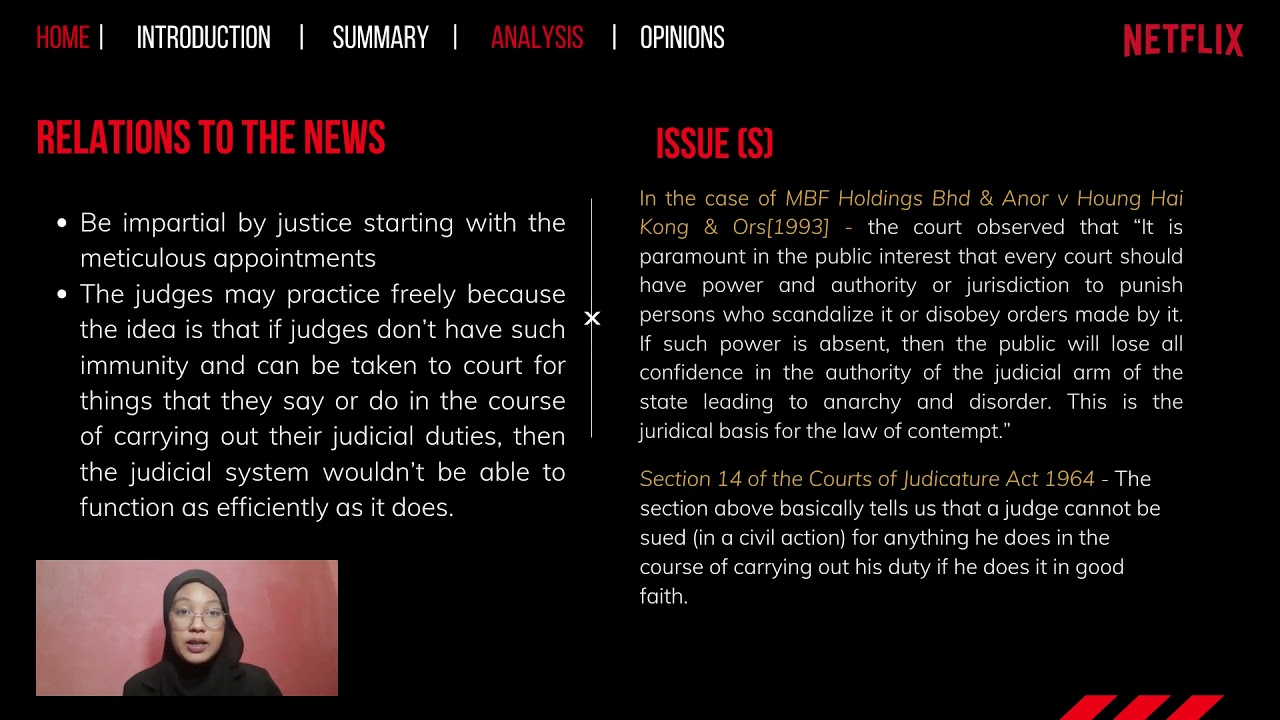The webpage features a sleek black background with navigation options in bold, uppercase text. At the top left corner, "HOME" is highlighted in red, followed by a white horizontal line. Adjacent to this, "INTRODUCTION" appears in white, then another white line, followed by "SUMMARY." Another white line leads to "ANALYSIS" in red, and finally another white line before "OPINIONS." 

Beneath these navigation items, "RELATIONS TO THE NEWS" is displayed in red, accompanied by a descriptive section with bullet points. Lower on the page, there is a medium pink rectangle showcasing a woman wearing a hijab and glasses, dressed in a black outfit.

To the right, a new section is demarcated by a vertical line with an "X" at its center, separating different headlines. Below this, the page discusses an "Issue(s)" followed by explanatory content. The bottom right corner of this section features three small diagonal red lines.